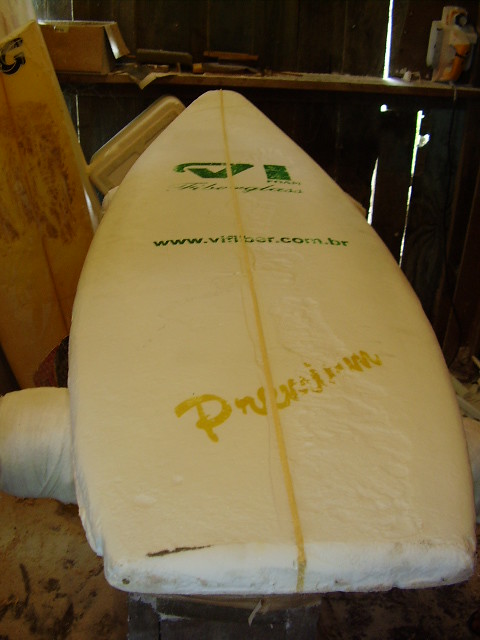This is a colored photograph taken indoors during daylight. It captures a white, short surfboard that could also be interpreted as a bodyboard. The board features a prominent yellow line running vertically down its center. At the top of the board, towards its pointed end, it displays green text with the letters "VI" and just below that, a partially legible URL that appears to be "viflfiber.com.br." Further down, in cursive yellow text, it says "premium," although the word is somewhat degraded. The board is housed within a wooden structure, likely a shed, visible through the slats and metal latch of a wooden door. The surfboard has a worn texture on the right side, indicating erosion of the wax.